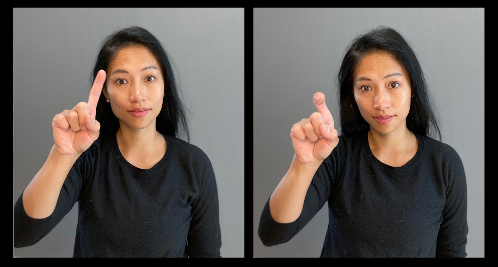This image features two side-by-side photographs of the same young Asian woman, possibly of East Asian, Vietnamese, or Filipino descent, standing in front of a gray wall. She has dark black hair and is dressed in a long-sleeved black shirt. Both images are outlined with a black border and a black line separates them. In the photograph on the left, she confidently holds her right hand in front of her with her index finger extended, as if indicating the number one or initiating a gesture. Her facial expression suggests she might be responding to a request or preparing to communicate. The image on the right shows her in a similar pose with the same background, but now her index finger is starting to curl down, suggesting a transition in her gesture. This shift hints at her possibly using or instructing in sign language, as her hand movements appear deliberate and expressive, despite the still image format making the precise context unclear.